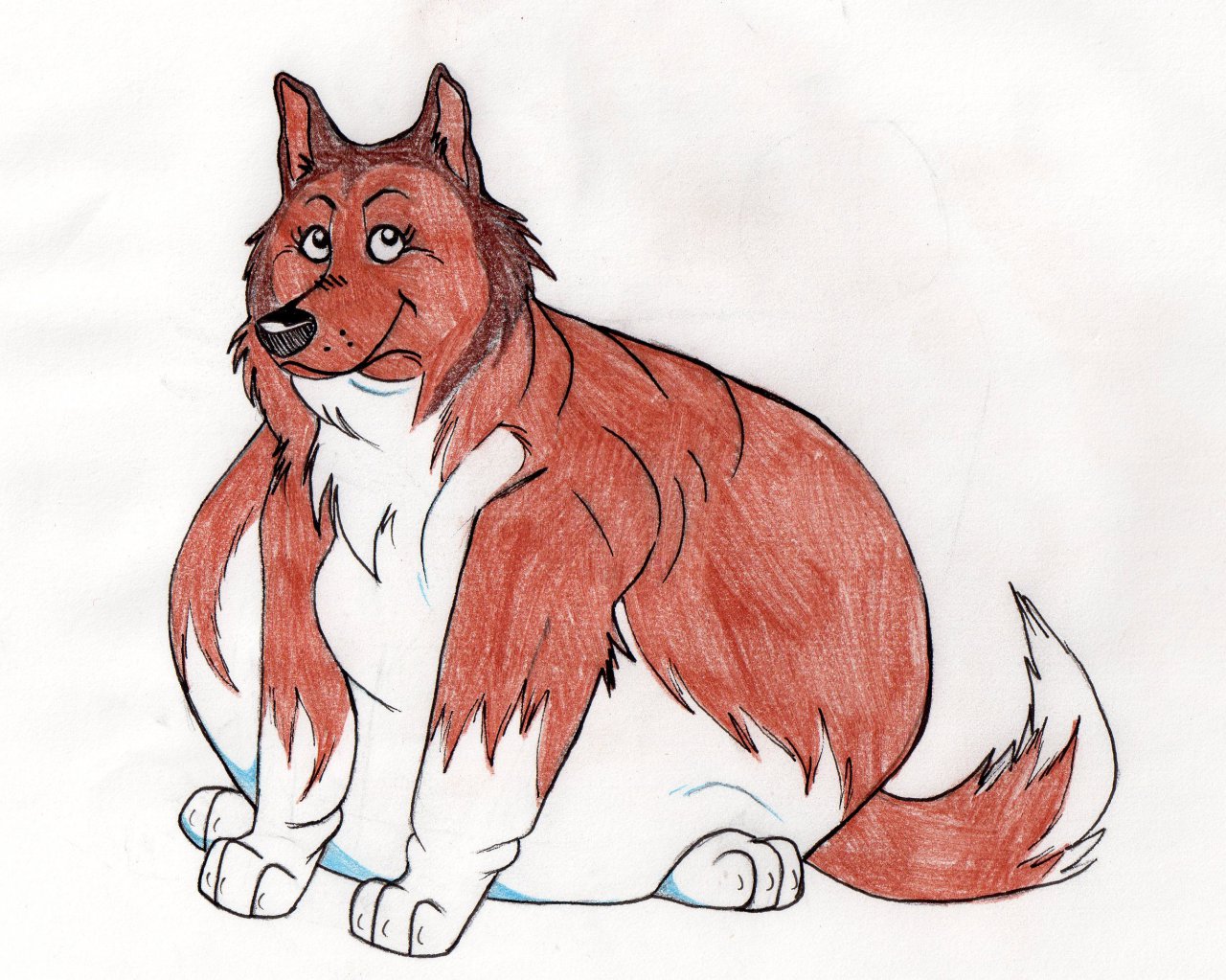This detailed drawing, created likely with medium-tipped markers or coloring pencils, depicts a chubby, rust-colored dog with a white underside and white-tipped paws. The dog's body is notably rounded and significantly larger than its head and legs, suggesting an overweight physique. It has a black nose and appears to be looking upward with a closed mouth, giving off a smug, content expression as if pleased with its condition. The tail transitions from red to white towards the end, adding to the charming aesthetic. The background is a simple off-white, with subtle hints of blue, emphasizing the vivid colors of the dog without any additional text or objects. This artwork captures a playful and endearing portrayal of an overweight dog, evoking a sense of humor and whimsy.